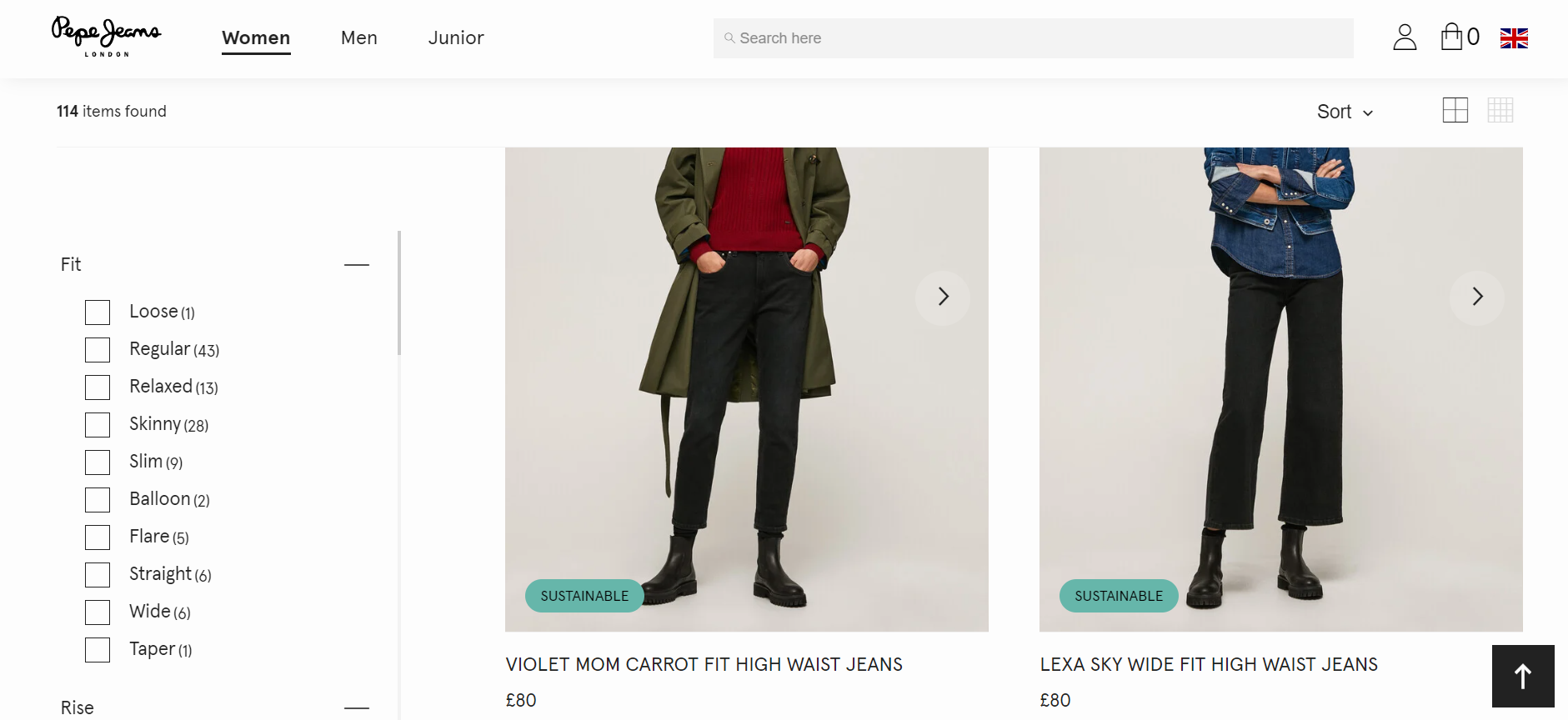Screenshot of the Papa Jeans website featuring three main categories: 'Women' (bolded and underlined), 'Men', and 'Junior'. On the left side, there is a filter section starting with the 'Fit' subsection, presenting a variety of fit options: loose, regular, relaxed, skinny, slim, balloon, flare, straight, wide, and taper. In the middle of the page, there are two prominent images of models showcasing the products. The model on the left is dressed in a trench coat paired with black jeans, while the model on the right sports a denim shirt or jacket with black jeans.